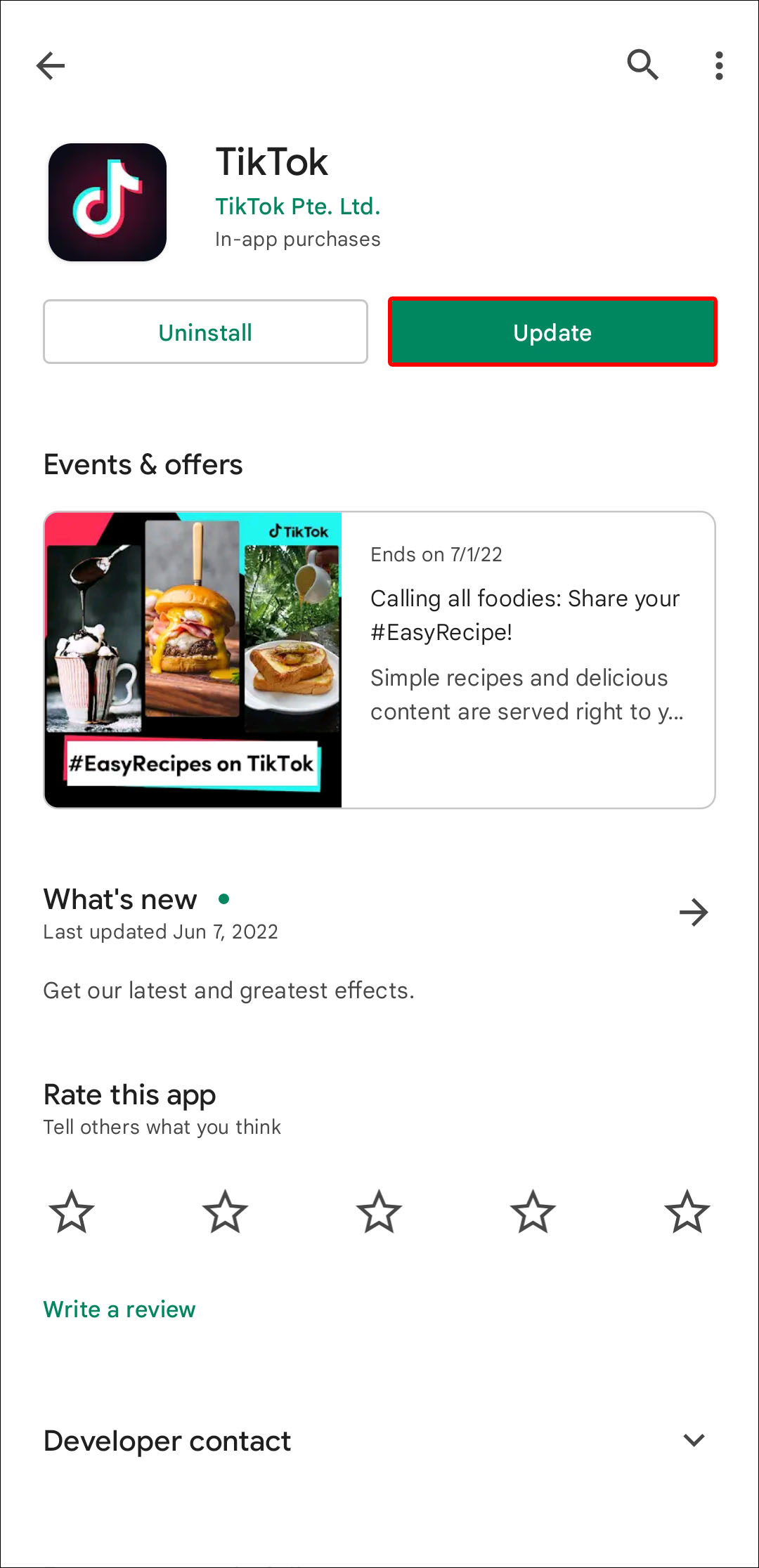The image is a screenshot from a mobile phone in portrait orientation, depicting the update screen for the TikTok app on the Google Play Store. At the top left, there's a back arrow, while the top right features a magnifying glass (search icon) and a vertical ellipsis (three dots) menu. On the upper left side of the screen is the TikTok icon, a small black square with a music note, followed by the text "TikTok" and "TikTok Pte. Ltd." indicating the app developer. Below this, it states that the app includes in-app purchases. 

Two prominent buttons are visible: "Uninstall" on the left and "Update" on the right. The "Update" button is green, indicating it has been selected. Below this section, in smaller black text, there's a portion labeled "Events and offers," highlighting a featured campaign called "Easy Recipes on TikTok." This section includes images of an ice cream sundae, a burger, and French toast, accompanied by the text "Calling all foodies, share your easy recipe" which is partially cut off, suggesting a call to action for user-generated content.

Further down, the screenshot displays the "What's new?" section, noting the last update on June 7th, 2022, with a brief mention of new effects being available in the latest update. This is followed by an invitation to "Rate this app" with five stars lined up horizontally, and an option to "Write a review."

Finally, at the bottom left, there is the "Developer contact" text with a downward arrow to its right, indicating a collapsible menu for contacting the app developer.